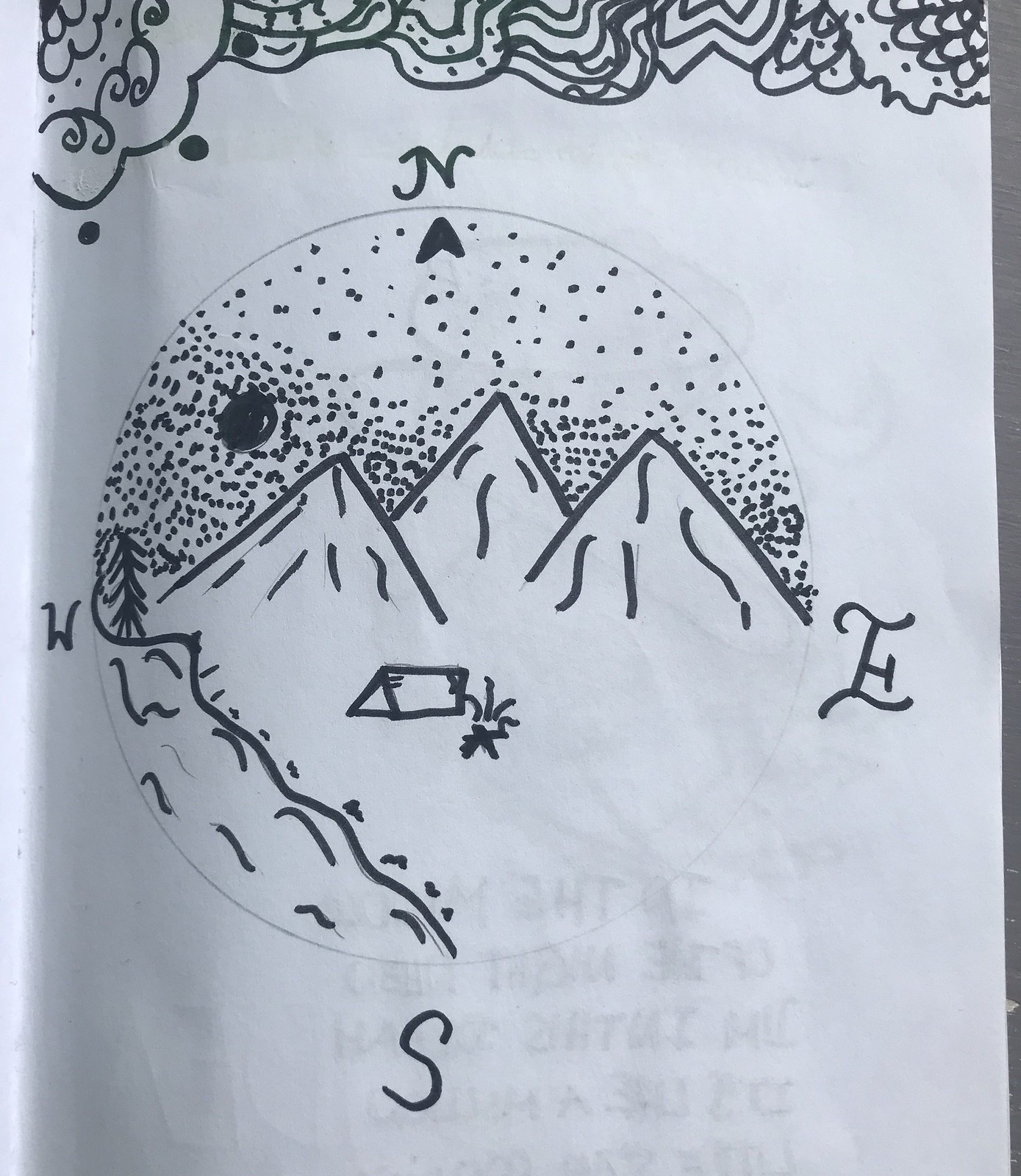The image appears to be a child's drawing executed on a white piece of paper using a black magic marker. The composition features a compass-like design with intricate details. At the top left-hand corner, there is a depiction of a sun, characterized by its scalloped edges and internal swirls. Surrounding the top portion of the drawing, various swirls add a decorative touch.

Central to the design is a large circle, faintly extending around the entire compass. Prominently displayed within this circle are ornate letters: an 'N' at the very top, an 'E' to the right, a 'W' to the left, and an 'S' at the bottom, each marking the cardinal directions.

The area around the top of the circle is adorned with small dots, transitioning to thicker dots positioned in the middle. These dots are set against a backdrop of three sharply pointed mountain peaks, each detailed with squiggly lines representing rugged terrain. Below the mountainous region, on the left side of the drawing, a river flows, complete with rippling effects to suggest movement. Nestled under the left-most mountain peak is a simplistic tent, accompanied by a small campfire, adding an adventurous, outdoor feel to the artwork.